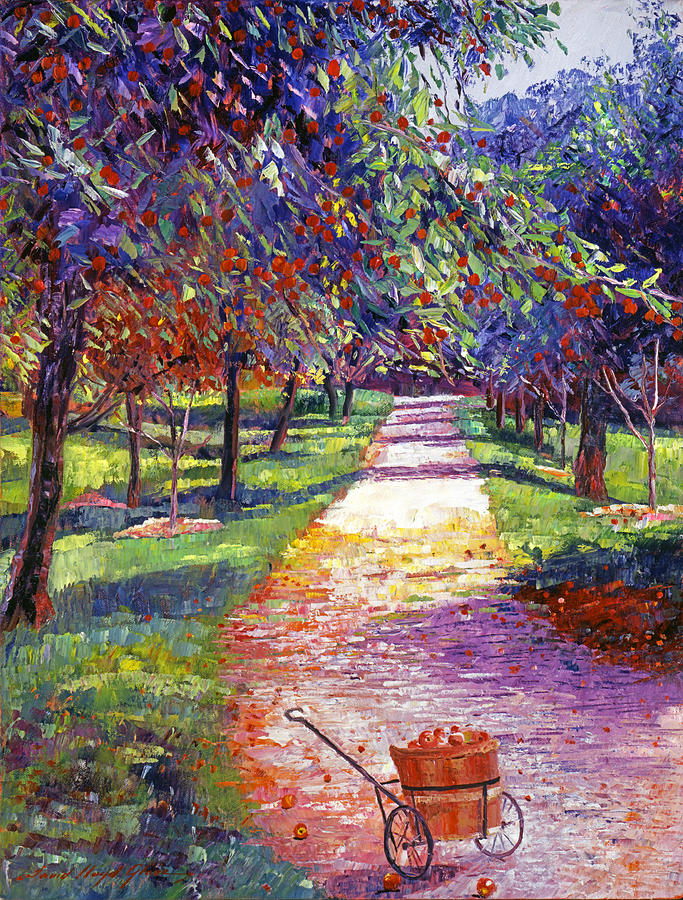The image depicts a vibrant, AI-created outdoor scene with an exquisite blend of colors that evoke an autumn ambiance. A winding pathway, adorned with shades of purple, orange, and white, stretches from the lower right corner, curves to the left, and continues straight through the center. Flanking the path are lush patches of green and blue grass interspersed with colorful shadows. Tall trees of varying hues, including red, green, and blue, line both sides, their leaves in the midst of transitioning to fall, some already scattered on the ground. 

In the lower foreground sits a quaint cart with two black metal wheels and a long handle, pointing towards the upper left. The cart carries a large brown wooden basket brimming with apples, some of which have tumbled onto the path, contributing to the rich tapestry of fallen leaves. Further into the scene, hints of bluish-white mountains emerge in the distant background, completing the picturesque landscape that exudes the tranquility of a serene morning.